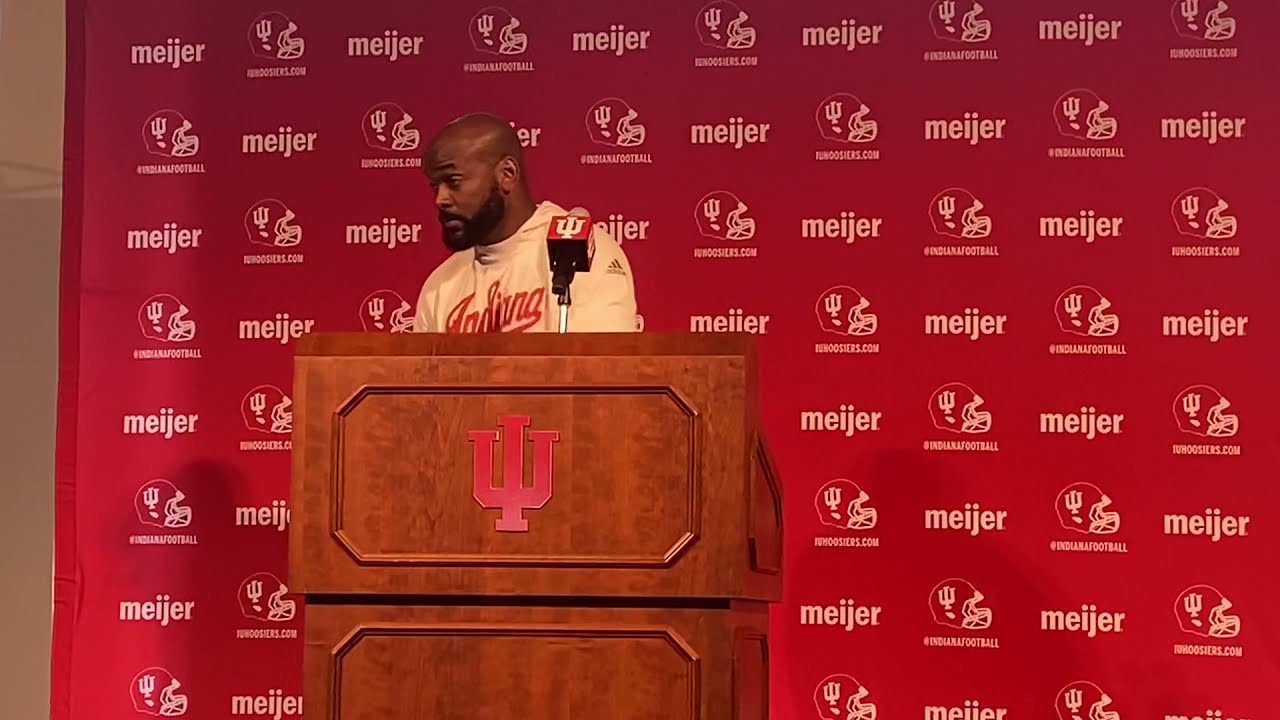In this image, a dark-skinned bald man with a thick black beard, likely a coach for Indiana University, stands at a wooden podium that bears the University of Indiana's logo, an interlocking "UI" in red. He is dressed in a light-colored, long-sleeve shirt with the Adidas logo and the text "Indiana" on it. The man is looking to his right, possibly listening to a question during what appears to be a post-game press conference. The background is a red banner that features alternating images of Indiana football helmets, the website indianafootball.com or handle @indianafootball, and the sponsor name "Meijer" (M-E-I-J-E-R). The scene suggests a formal media setting following a sporting event, with the man appearing to be introspective or possibly disinterested.